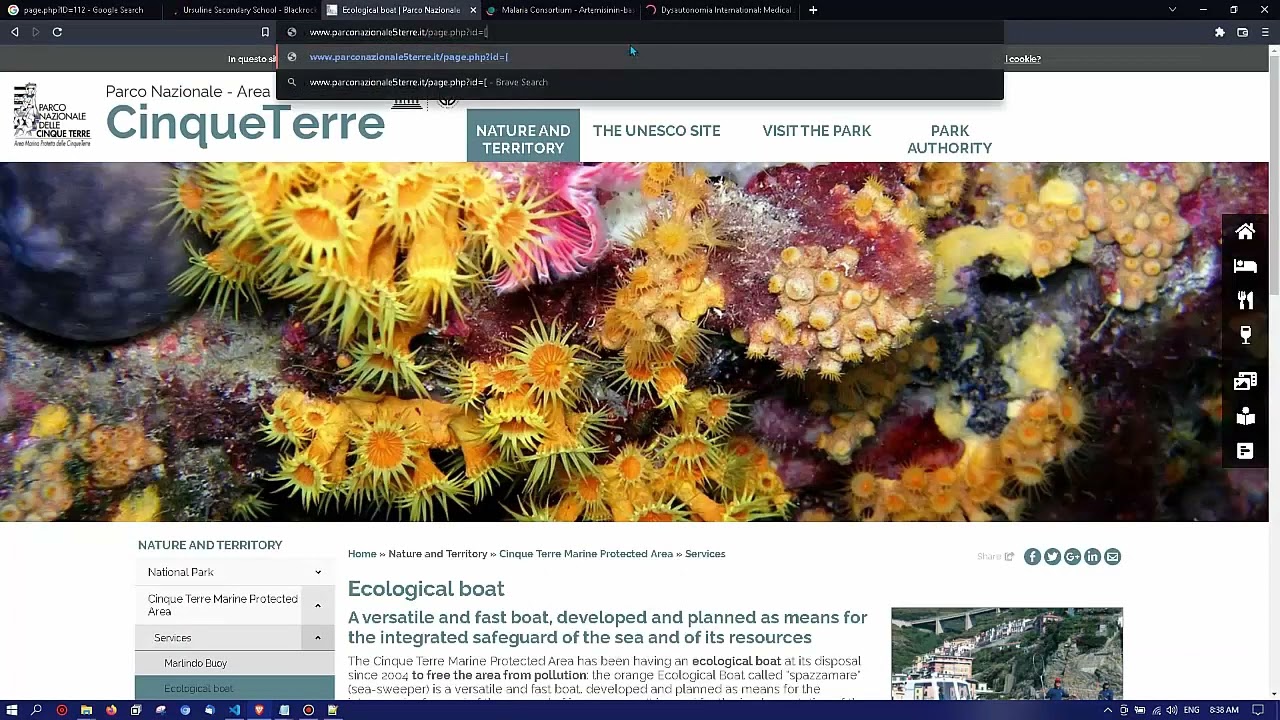The image showcases a webpage with a distinct layout. At the top, there is a black banner containing small, somewhat blurred text that is difficult to read. Below the banner, two tabs are visible on the browser. The web address is displayed in blue print, accompanied by a black dropdown menu that overlaps a white banner. The white banner features the text:

"Parco Nazionale del Cinque Terre" (P-A-R-C-O-N-A-Z-I-O-N-A-L-E and C-I-N-Q-U-E-T-E-R-R-E), followed by phrases like "Nature and Territory," "The UNESCO Site," "Visit the Park," and "Park Authority."

Descending further, a graphic is depicted, likely showing flowers or possibly sea plant life. Below this graphic, additional text reads:

"Nature and Territory,
National Park Services,
Malindo Bay Ecological Boat."

This section continues with a detailed description of the ecological boat:

"A versatile and fast boat developed and planned as a means to integrate and safeguard the sea and its resources."